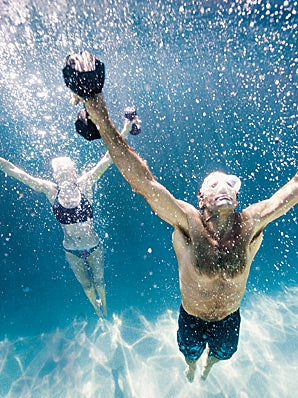The photograph captures a slightly blurry underwater scene in a swimming pool featuring two individuals. Both the man and the woman are positioned vertically with their hands raised, each holding a circular object that appears to be a weight, black on either end. The woman, situated on the left, wears a black swim top and blue bikini bottoms. On the right, the man sports black shorts and transparent goggles. They are surrounded by numerous shimmering white bubbles rising through the blue water, with light scattering at the bottom of the image, adding a subtle glow to the scene.